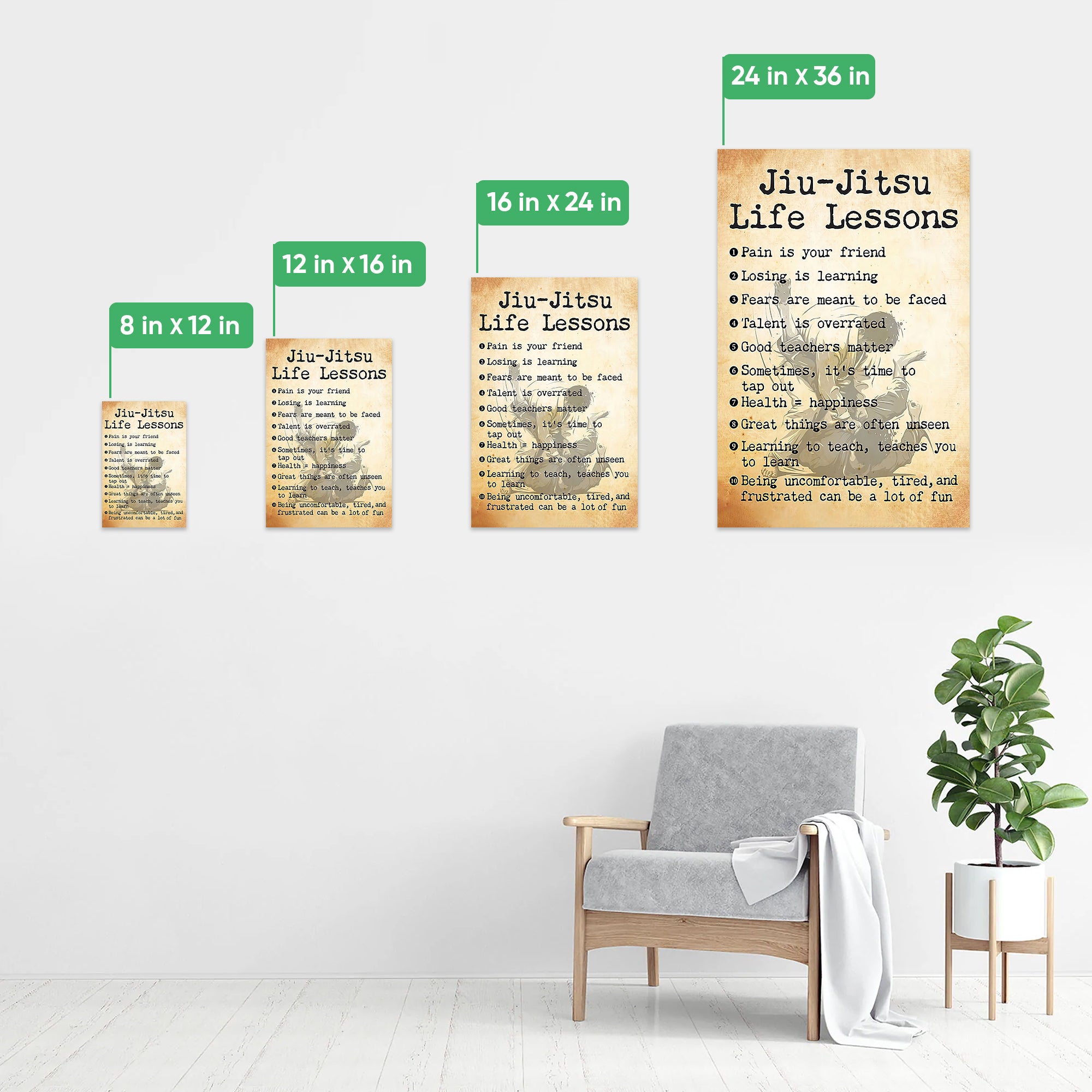The image depicts a neatly arranged room with white tiled flooring and an off-white wall adorned with four differently-sized posters displaying Jiu-Jitsu Life Lessons. From left to right, the poster sizes are 8x12 inches, 12x16 inches, 16x24 inches, and 24x36 inches. Each poster features the same beige parchment texture with black text, and they all have green flags indicating their dimensions. The text on the posters reads "Jiu Jitsu Life Lessons" at the top, followed by ten numbered bullet points that include phrases like "pain is your friend", "losing is learning", "fears are meant to be faced", and "talent is overrated", among others.

In the lower right corner of the image, there is a comfortable gray-cushioned chair with a light wooden frame, wooden armrests, and legs. A white towel is draped over the chair's left arm, extending down to the floor. To the right of the chair, there is a potted plant with large green leaves, slightly taller than the chair itself. The plant is housed in a white planter elevated by a wooden stand with four legs. The overall arrangement creates a cozy and motivational atmosphere, combining elements of comfort and inspiration.